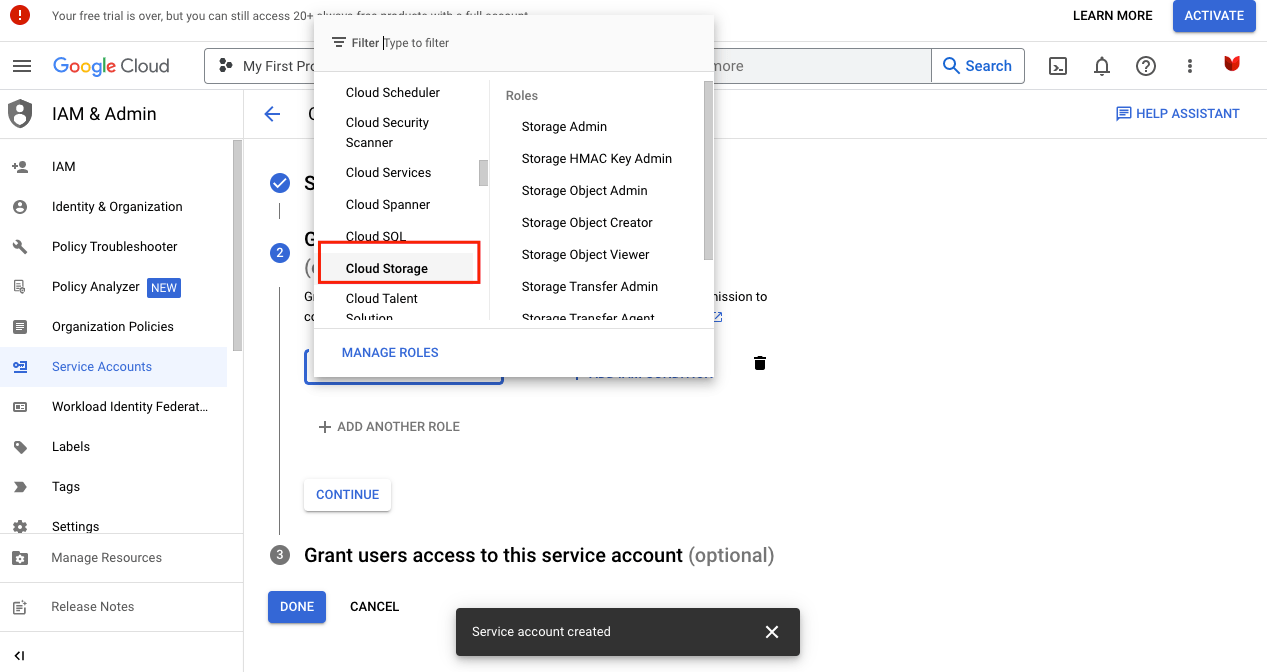**Detailed Caption:**

This landscape-oriented photo captures a section of a Google Cloud page. The top of the page features a horizontally-aligned thin gray border resembling a title bar. Above this border, prominently displayed, is a red circle with a white exclamation mark inside it, accompanied by the text, "Your free trial is over. You can still access 20+," although the rest of the text is cut off. To the right of this alert, situated in the corner, there are clickable elements: a "Learn More" link followed by a blue "Activate" button with white text.

Below the title-like area, the layout resembles that of a Google Mail interface. On the left side, there's a hamburger menu icon beside the Google Cloud logo. Directly beneath the logo, there is a shield icon labeled "IAM & Admin" which is followed by various options including IAM, Identity and Organization, Policy Troubleshooter, Policy Analyzer, and additional items.

To the right of the Google Cloud menu, there is a search box featuring a gray background and gray placeholder text, with the actual search field having a white background. The blue magnifying glass icon and the word "Search" are also highlighted in blue. Adjacent to the search box are several icons: a user photo icon, a notification bell icon, a question mark icon, and other icons that are not clearly visible.

Further down, there is a link labeled "Help Assistant" in blue. The main body of the page is set against a white background, displaying what appears to be a partially visible process or task list. This section is obscured by a pop-up box presenting various options, with "Cloud Storage" highlighted in red.

**End of Caption**